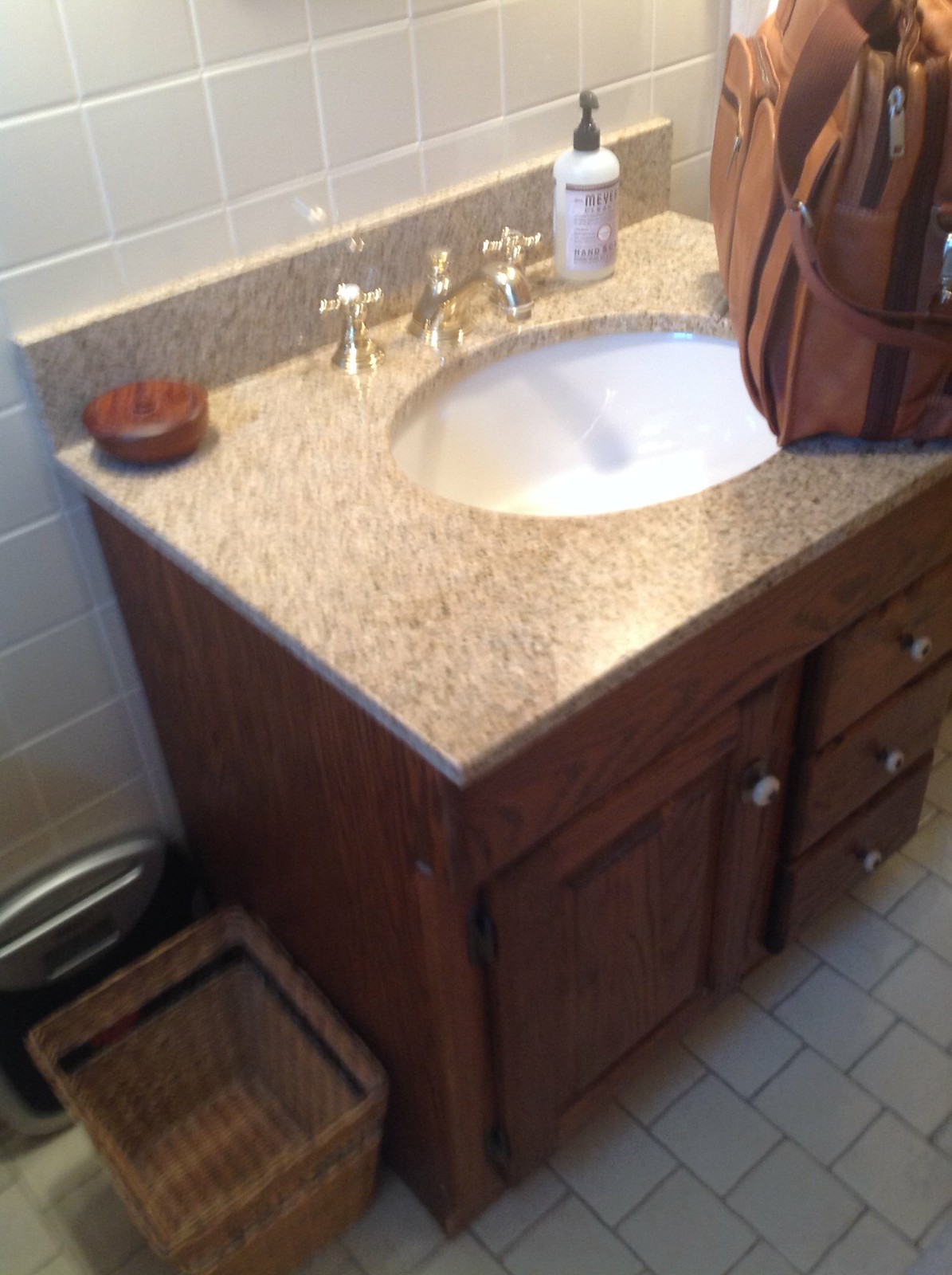In this detailed photograph of a bathroom, the floor is adorned with dark, light beige ceramic tiles, which create a warm and inviting atmosphere. Covering the walls, there are also ceramic tiles, but in a much lighter shade—either light gray or light beige—adding a touch of elegance and contrast to the space.

The focal point of the image is a stylish bathroom vanity cabinet crafted from dark-finished wood. The cabinet features a door and three drawers, offering ample storage space. Topping the vanity is a countertop that exudes sophistication with its textured, speckled finish, resembling gray granite.

Perched on the countertop is a compact leather backpack or travel bag, made from rich, brown leather. Adding a touch of luxury to the vanity is a widespread faucet, finished in gleaming gold or brass.

On the floor, next to the vanity, a square wicker basket provides additional storage. Leaning against the wall behind the basket is a modern, black and gray scale, ready for use. Enhancing the hygiene and aesthetic of the vanity is a hand soap dispenser with the brand name "Meyer" clearly readable on its label. This detailed setup combines functionality with a sophisticated design, creating a comfortable and stylish bathroom space.